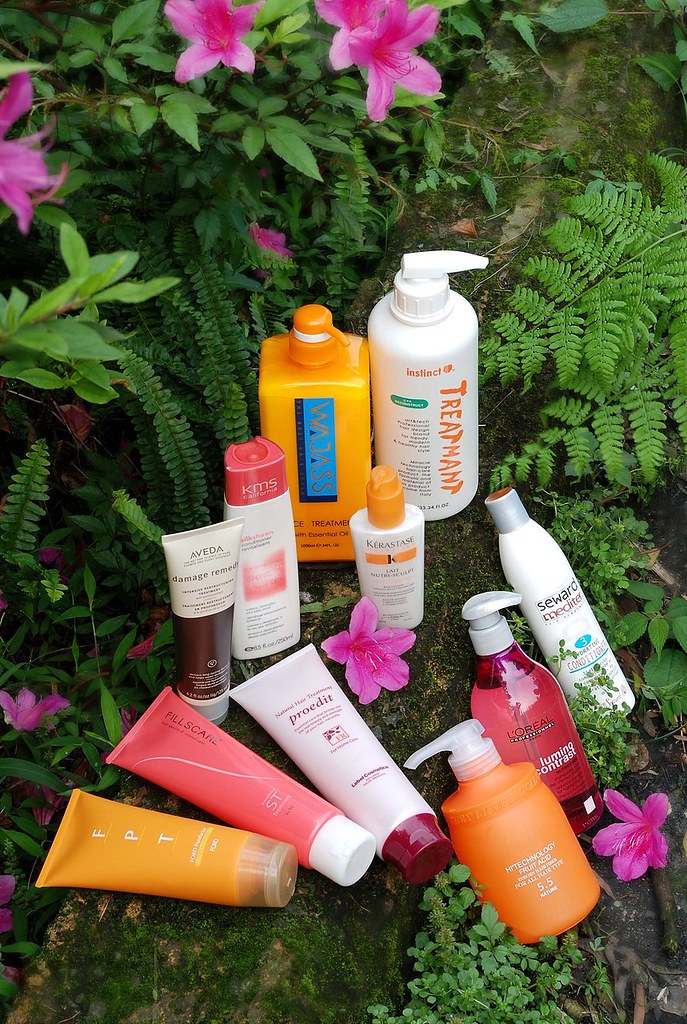A vivid, brightly photographed image of assorted body products displayed against a lush, green backdrop of fronds and vibrant purple flowers. The colors in the image are highly saturated and rich, enhancing the visual appeal. A moss-covered log diagonally crosses the frame from the bottom left to the top right. The image, which is taller than it is wide, features various beauty products arranged artistically on the log. 

On the top of the log sit two bottles: one orange and one white. Just below them are two more bottles, one with a red cap and the other with an orange cap. Following them is a brown and white product. Further down the log, three bottles lie on their sides. The text on these bottles reads "ProEdit," "PhilSkafic," and "FTP." 

Finally, on the right side of the log, three additional products lean against it: one appears to be an exfoliant or fruit-based dispenser, another is a L’Oreal product labeled "Luminating Contrast," and the third resembles a Mediterranean-inspired shampoo container. The meticulous arrangement and vivid presentation make this image an eye-catching display of beauty products.